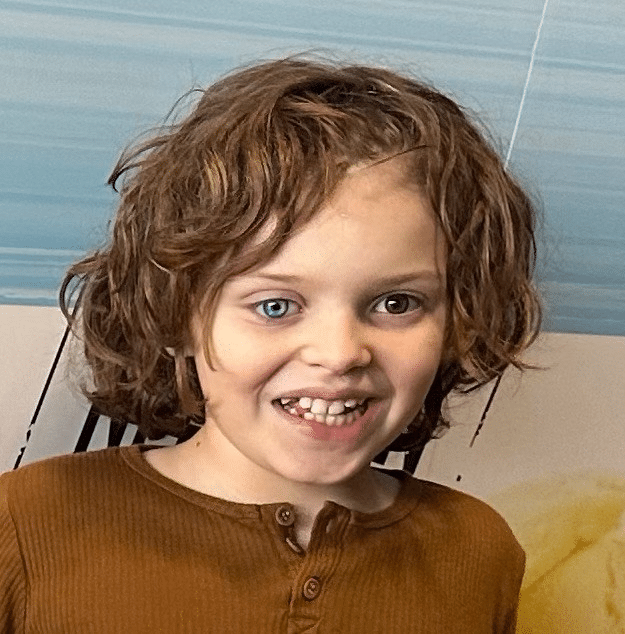The photograph features a young child with striking heterochromia, displaying one blue eye and one brown eye. The child has chin-length, brown, curly hair that frames a beaming face filled with a youthful, excited expression. Their smile showcases straight white teeth, with some gaps indicating the process of losing baby teeth and growing new ones. The child is dressed in a henley top, rust-brown in color, with three buttons at the collar. Set against a background with blue aluminum window shades at the top and white tiles below, the scene suggests the child might be seated on a taupe-colored couch. Off to the left, there appears to be a yellow towel. The combination of the child's distinctive eyes, playful smile, and charming attire creates an engaging and memorable image.